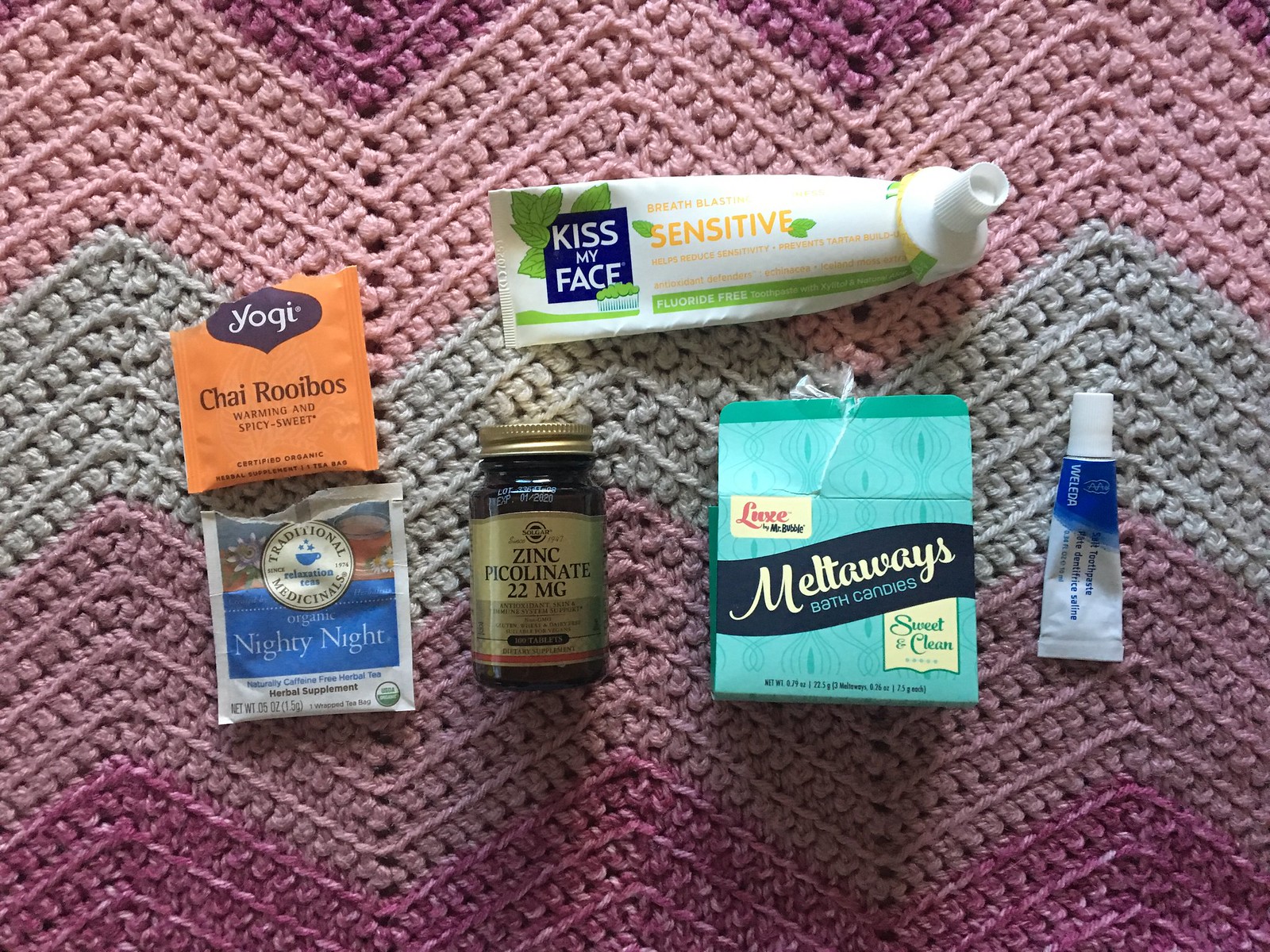This photograph captures a variety of objects meticulously arranged on a knitted blanket that flaunts a gradient of purples and blues. The blanket's intricate design features alternating peaks in shades of rich dark purple, light purple, a delicate light blue, and then transitioning back to a deeper purple hue towards the top. 

Among the objects displayed, there is an orange square package adorned with a blue accent at the top and inscribed with the text "Yogi" and "Chai Rubios" in bold black lettering. Positioned beside it is a tube of cream, predominantly white with blue and green highlights, exuding a sense of medical or cosmetic purpose. A similarly sized blue and white square box nearby reads "Nighty Night" in prominent white letters. 

Additionally, a small brown and gold bottle labeled "Zinc Picolinate" is included in the assortment, suggesting a nutritional supplement. Adjacent to this bottle, there's a square box with a soothing light blue and dark blue palette, marked with the name "Meltaways" in distinct white text. Lastly, a petite vertical tube, predominantly blue with white accents, completes the collection, contributing to the diverse array of items meticulously presented on the beautifully woven backdrop.